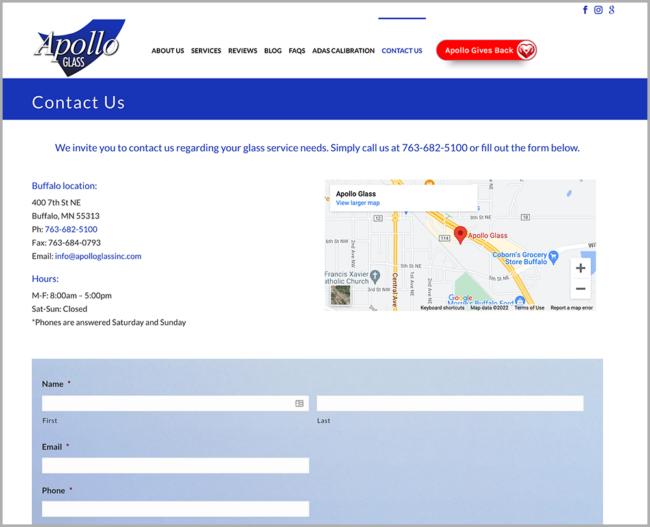The website screenshot of Apollo Glass features the company logo prominently positioned at the top left corner. The logo consists of the text "Apollo Glass," presented in a distinct font: "Apollo" is in a large, white-yellowish font with "Glass" in a smaller, centered font directly beneath it. Behind the text "Apollo," there is a large, blue ribbon-like check mark, adding a unique visual element to the logo.

The website has a clean, white background and a menu bar at the top that includes sections titled About Us, Services, Reviews, Blog, Facts, and Contact Us. There is a notable red button labeled "Apollo Gives Back," adorned with a heart icon, suggesting a charitable or community-focused initiative by the company.

The screenshot appears to be taken from the Contact Us section of the website, specifically showing details about the Buffalo location in Buffalo, Minnesota. Another section labeled "ADAS Calibration" is also visible, indicating one of the services offered by Apollo Glass.